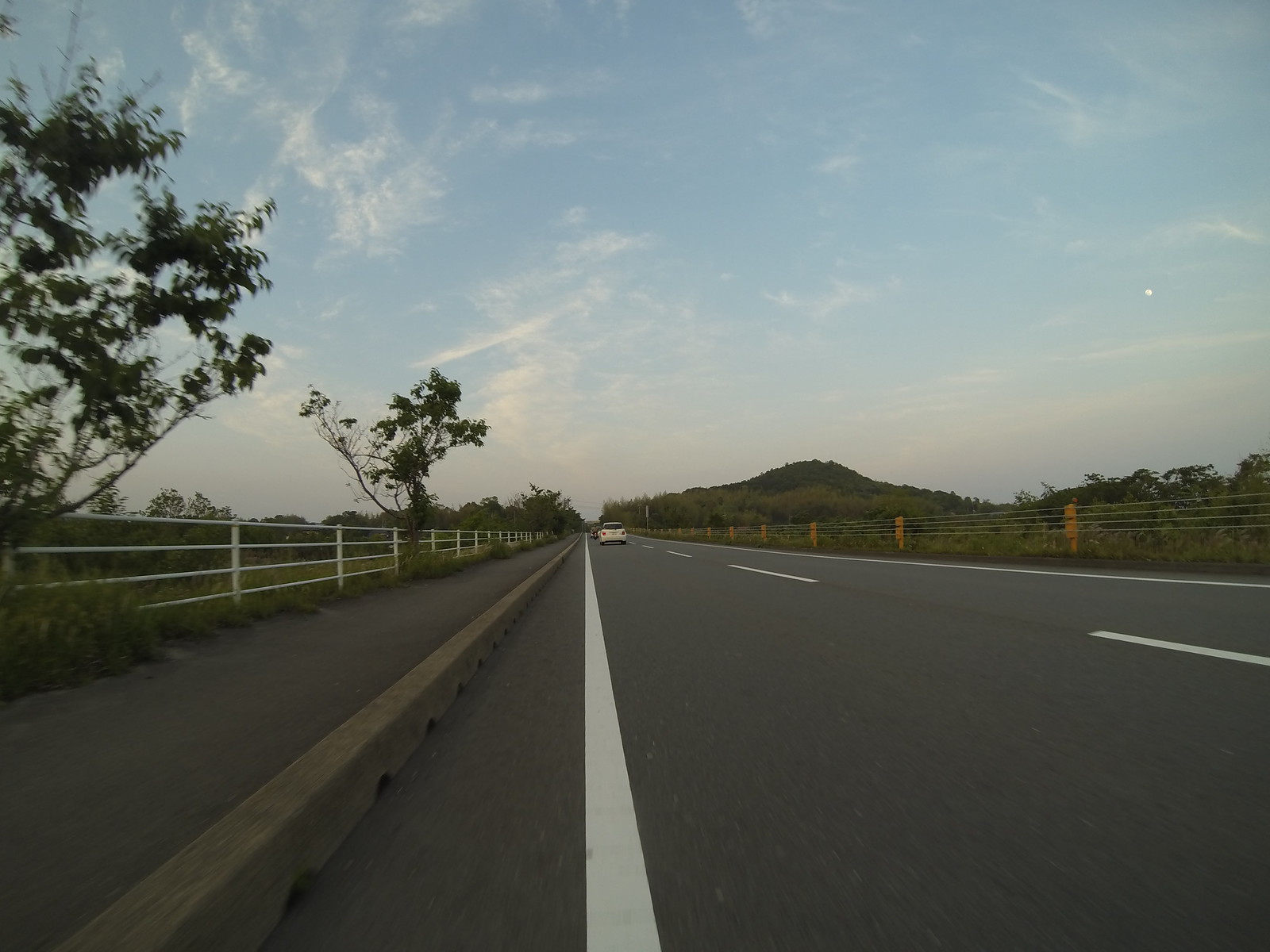A serene, early morning or dusk scene captures a car traveling away from the viewer on a recently paved two-lane road, its taillights glowing red as it heads towards a gently sloping green hill in the distance. The smooth asphalt road is flanked by a solid white line extending from the bottom center of the image towards the middle, which eventually meets the horizon, creating a sense of infinity. The lower left-hand third of the image features a low concrete barrier running parallel to a white metal fence, which is accompanied by scattered trees and greenery. On the right-hand side, another metal fence with different posts lines the road, bordering grassy areas interspersed with bushes. The upper portion of the rectangular frame showcases a blue sky adorned with delicate wispy clouds, and an almost discernible moon hangs faintly on the right, completing the tranquil outdoor setting.